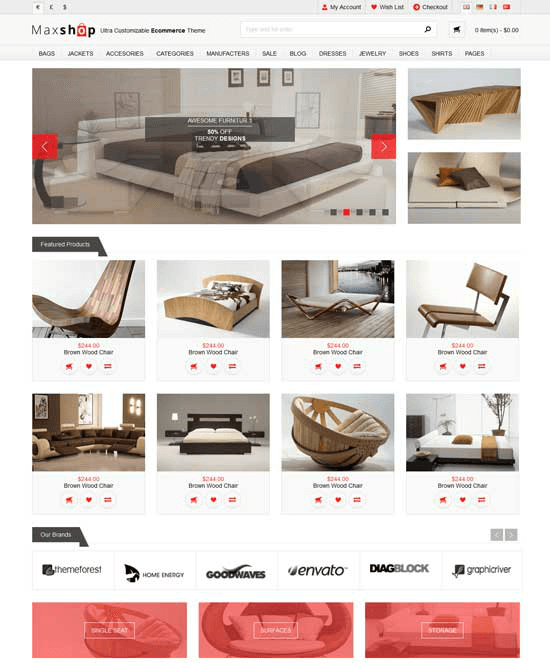This image is a screen capture from a computer monitor displaying the home page of a furniture shopping website called "Mac Shop." Located in the top left corner, “Mac Shop” is written in gray and black lettering, with the ‘O’ replaced by an orange shopping bag featuring a white 'O'. Adjacent to this, in the header, the phrase "Ultra Customizable E-Commerce Theme" is displayed.

The top right corner showcases a series of navigational buttons, each adorned with an orange icon. From left to right, these buttons include "My Account" (represented by a person icon), "Wish List" (indicated by a heart icon), and "Checkout" (depicted with a down arrow icon). On the far right, there are three very small square icons whose specific functions are unclear due to their size. 

Below this row, a white search bar with a gray magnifying glass icon is situated, followed by an unusual gray design on a white square button. The main navigation bar spans across the top of the page and is highlighted in a gray strip, featuring site labels from left to right: "All in Black," "Bags," "Jackets," "Accessories," "Categories," "Manufacturers," "Sales," "Blog," "Dresses," "Jewelry," "Shoes," "Shirts," and "Pages." Notably, despite these categories suggesting apparel and accessories, the page content is exclusively focused on furniture.

The top section prominently features a wide image slideshow option showcasing a contemporary king-size bed. To the right, there are two smaller stacked images displaying an unconventional table. Below, the next row includes images of various wooden furniture items: a chair, a bed, a lounge-type cot bed, and a modern office chair, all in shades of brown. 

Following this, there's another row presenting a curvaceous sectional sofa, a multi-section sofa, a dark Asian-style ebony double bed, a basket-style brown chair with a white cushion, and another bed with white and gold sheets. Each furniture piece is labeled with its name and price point, accompanied by three round icons below each image: an orange heart (likely for the wish list), a small shopping bag, and an unspecified third icon.

At the bottom of the page, three red-hued images are semi-transparently overlaid with white square identifiers. Centered above these images are logos representing various companies: ThemeForest, Home Energy, Good Waves, Envato, Diagblock, and Graphdriver, listed from left to right.